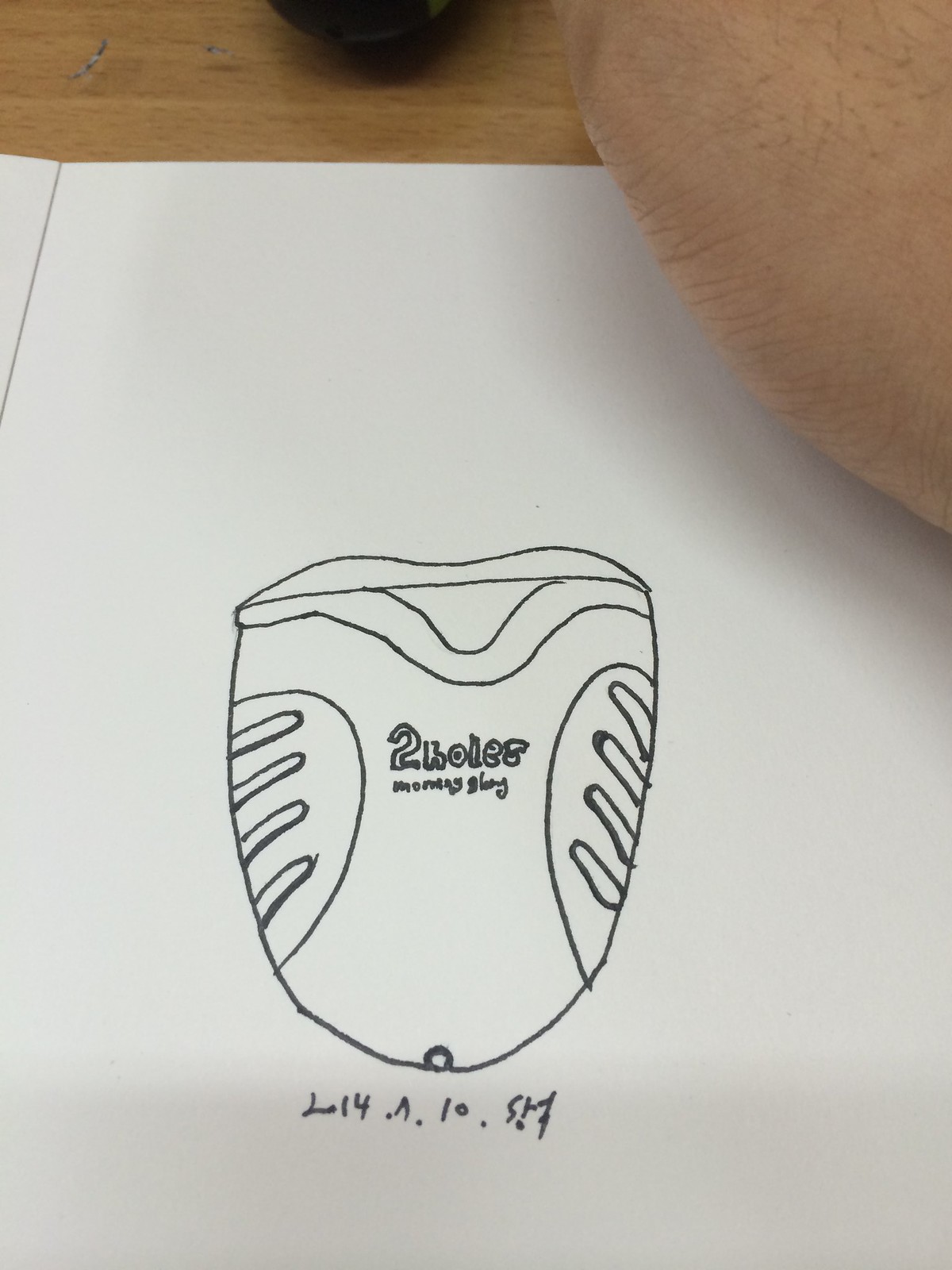The image depicts a black fine-tipped marker sketch of an object on white paper, possibly a computer mouse or an AirPods case, drawn in a sketchbook on a wooden table. The sketched object is semi-oval and somewhat shield-shaped, featuring four notches along its curved sides. The upper section has wavy borders, and it includes the text "2 holes" prominently written across it. Additionally, there is fine, largely illegible text beneath, which seems to read "morning sky" or something similar. At the bottom, there are ambiguous letters and numbers such as L14, 1.10.SM or L.14.A.10.SNQ. In the upper right corner of the image, there's a slightly out-of-focus close-up of a relatively hairy Caucasian hand or elbow, likely belonging to the person who drew the sketch.